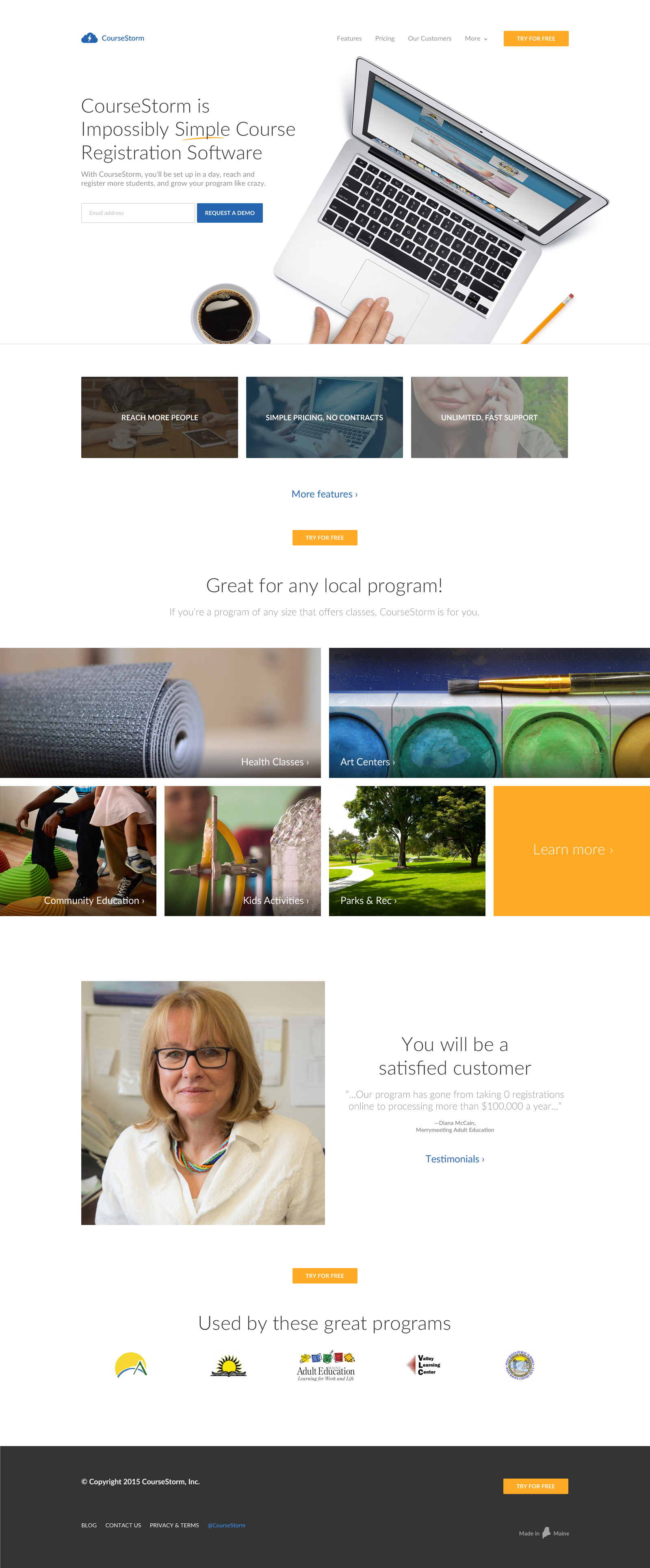Here is the cleaned-up, detailed caption for the image:

This screenshot showcases a webpage viewed on a phone. In the top-left corner, there's a logo that is hard to decipher. The header contains five links, with the fifth one being a prominent yellow button. Below the header, an image depicts a laptop with a person's hand on the trackpad, accompanied by the text "CourseStorm is impossibly simple course registration software." A small blurb follows, though it's too small to read clearly. Further down, there's a text box labeled "request a demo," likely for email input, accompanied by a blue button. Below this, three clickable images are displayed, each highlighting different features: "reach more people," "simple pricing, no contracts," and "unlimited fast support." A "more features" button and another illegible orange button are present. The webpage emphasizes various local programs such as health classes, art centers, community education, kids' activities, and parks and recreation. There's also a section titled "testimonials" featuring a picture of a blonde-haired woman wearing glasses with an assurance of customer satisfaction. Another orange button with unreadable text concludes the page.